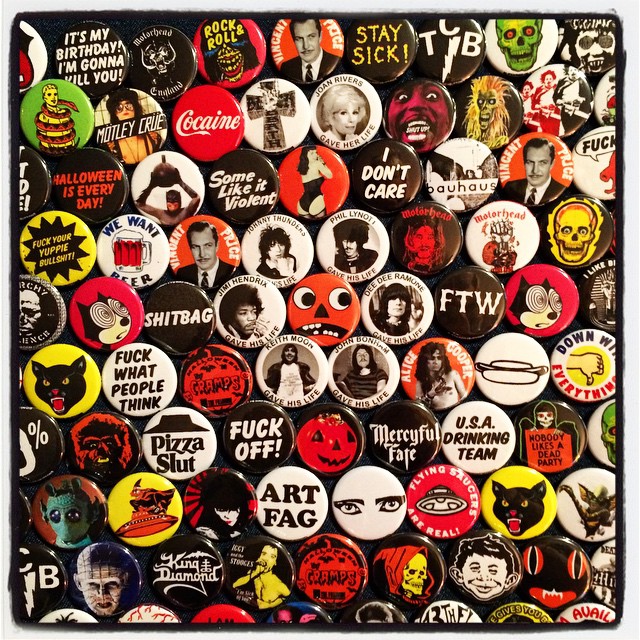A collection of dozens of small, round buttons, each featuring various images and phrases, is arranged on a blackboard with rounded corners, forming a square shape. The buttons are the type you pin to your shirt and are adorned with designs spanning music, movies, and counterculture themes. Notable buttons include several with negative or rebellious messages such as "It's My Birthday, I'm Gonna Kill You," "F*** What People Think," "F*** All," "S*** Bag," and "USA Drinking Team." 

Icons such as a yellow button with a black panther with gold eyes and red facial features, and a vintage Pizza Hut button also stand out. Specific imagery includes a Motorhead logo, a Vincent Price portrait, a green skull, the Kramps logo, and a cross within a white circle. There are multiple horror-themed buttons like one featuring Pinhead from Hellraiser and another with the Texas Chainsaw Massacre logo. A red figure exclaims "Shut Up," and a button declares "Halloween Is Every Day" in red font. The collection also features pop culture icons such as Betty Page in red, a model that resembles Joan Rivers with the text "Joan Rivers Gave Her Life," and a tribute to Dee Dee Ramone.

Amidst the mix are pins stating "Still Sick," "Some Like it Violent" in black and white, "Art Fag," "CF Off," "Merciful Fate," "FTW," and "I Don't Care." Among this colorful array, there's a mix of a skeleton head, a cartoon rat, and instances of Freddy Krueger and Jason imagery. Overall, these buttons paint a vibrant, albeit edgy, display of personal expressions and cultural references.